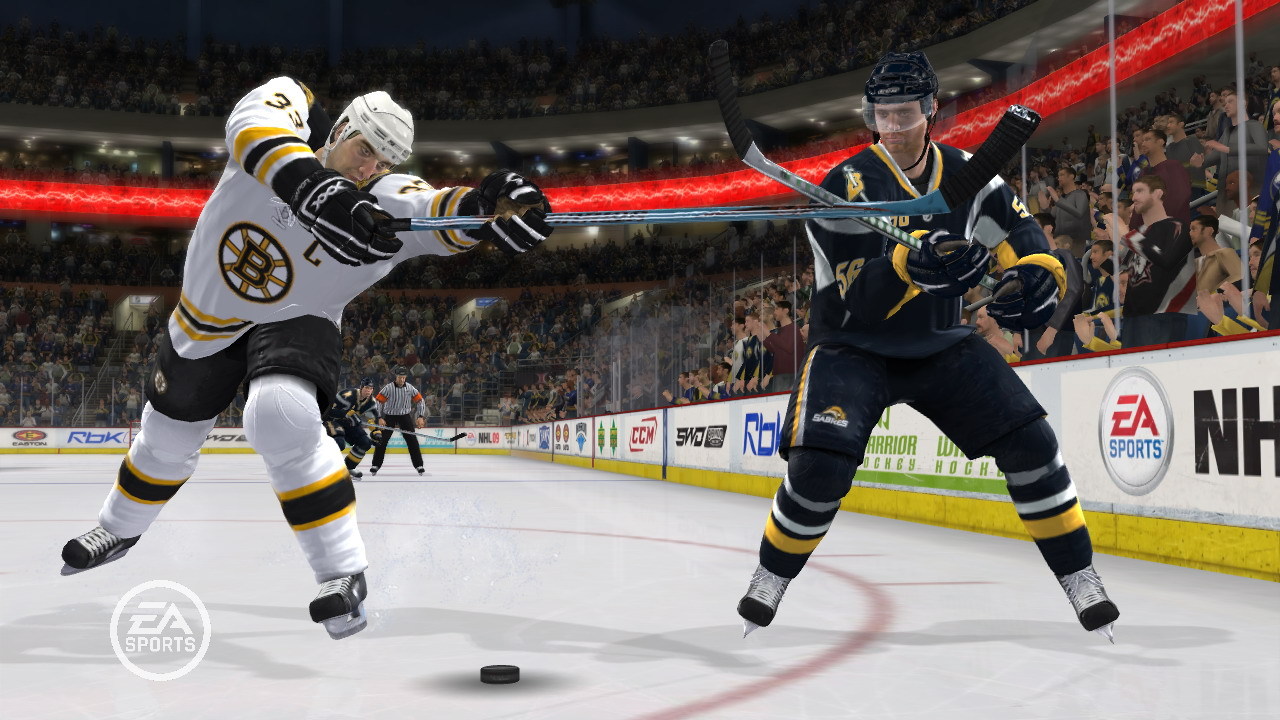In this dynamic hockey scene, two players are captured in an intense moment on the ice. On the left side of the image, a Boston Bruin is in action, donned in a white jersey contrasted by black shorts and white leggings featuring a black and gold band around the calf. His uniform is accessorized with a white helmet and black and gold padding on his forearm. Positioned with his right leg extended behind and his left leg bent forward, he reaches out with his hockey stick towards an opposing player.

The other player, situated on the right side of the image, is dressed in an all-black uniform accented with white and yellow bands around the legs and forearms, and a touch of yellow around the neck. His legs are spread apart, and he uses his stick to intercept the Boston Bruin's reach. Between them, the puck lies on the ice, adding to the tension of the moment.

In the background, a crowd of spectators is visible, gathered near the edge of the rink. A distinct curved red line marks the rink’s boundary, extending from the upper left-hand side and sweeping across before exiting the frame in the upper right corner. The upper background is notably dark, highlighting the vibrant action on the ice below.